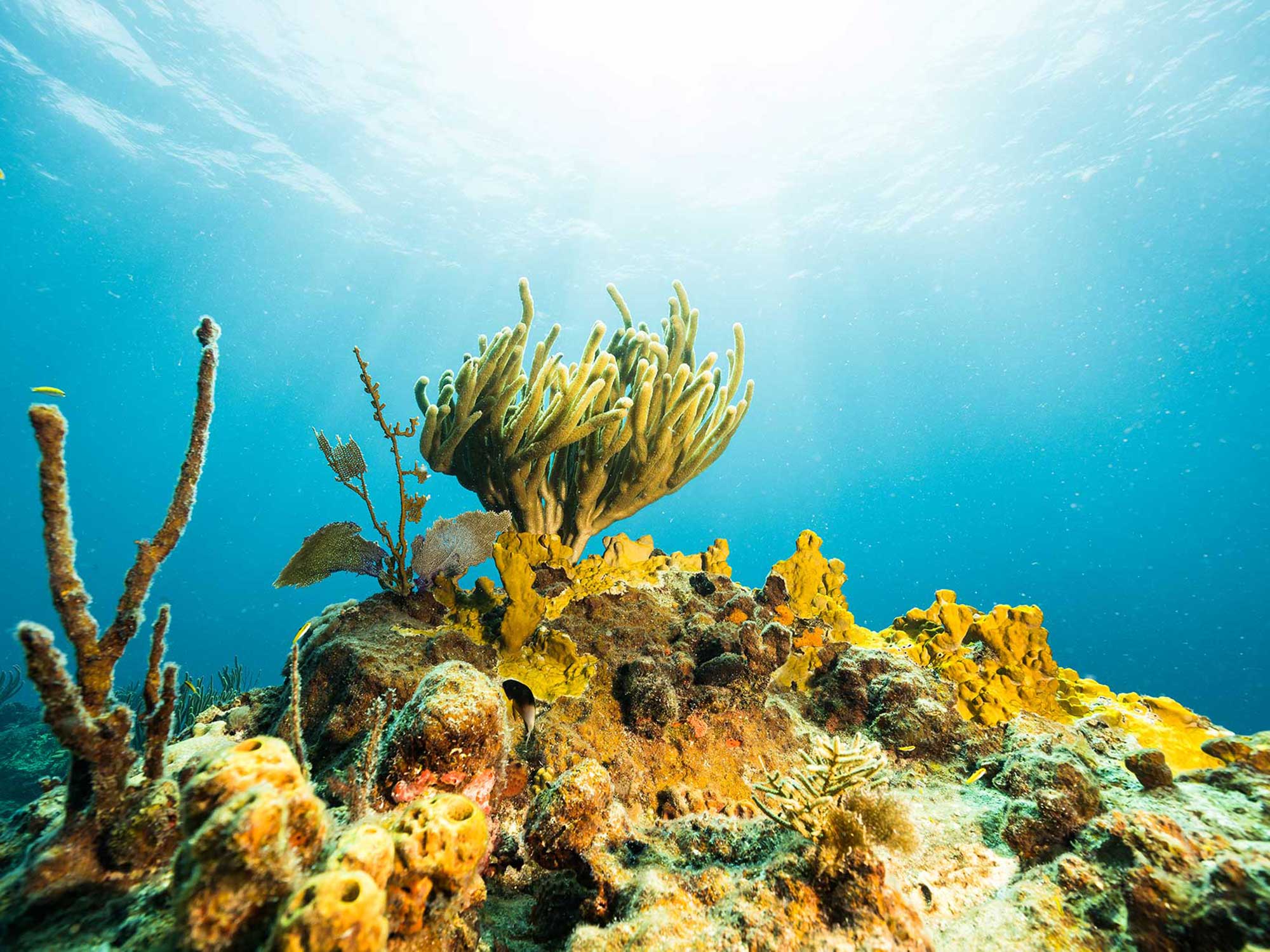The photograph captures a detailed underwater scene of a coral reef bathed in sunlight filtering through the water from above. The coral reef, situated at the bottom and center of the image, showcases a variety of coral types including light brown, yellow, and touches of beige, green, orange, pink, and brown hues. The corals exhibit numerous textures, with some resembling rocks, others appearing finger-like or resembling sea anemones, and a distinctive piece with tentacles at the top center of the reef. Although marine life is sparse, a few small fish can be spotted, including a yellow fish and a black fish. A tall, thin piece of coral resembling a stick stands out on the left side of the photograph with a small fish positioned just above it. The overall scene is well-lit, casting a question on its realism due to the pristine illumination, adding a surreal quality to this underwater tableau.